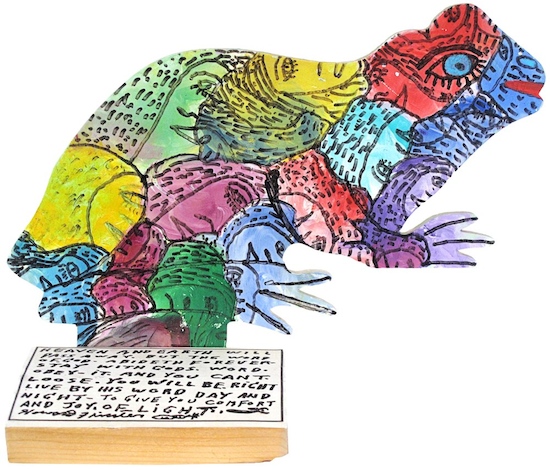This detailed and vivid artwork, titled "Frog," was created by Howard Finster in 1995. The piece, set in a landscape orientation, portrays an abstract, colorful frog. The vibrant frog or chameleon figure features an eclectic blend of colors including reds, blues, purples, yellows, and greens, with intricate black stripes or dots accentuating various parts of its body. It boasts distinctive blue eyes, a red mouth, and outstretched fins, with human half-faces creatively integrated throughout its form. The reptile-like figure displays a fascinating mixture of claws and a smile, further enhancing its whimsical nature. In the foreground, adjacent to the frog’s back leg at the bottom left corner, lies a stack of cards with handwritten text in black, though the phrases are largely illegible. This piece, embodying the art brut style, is a compelling example of modern folk art.